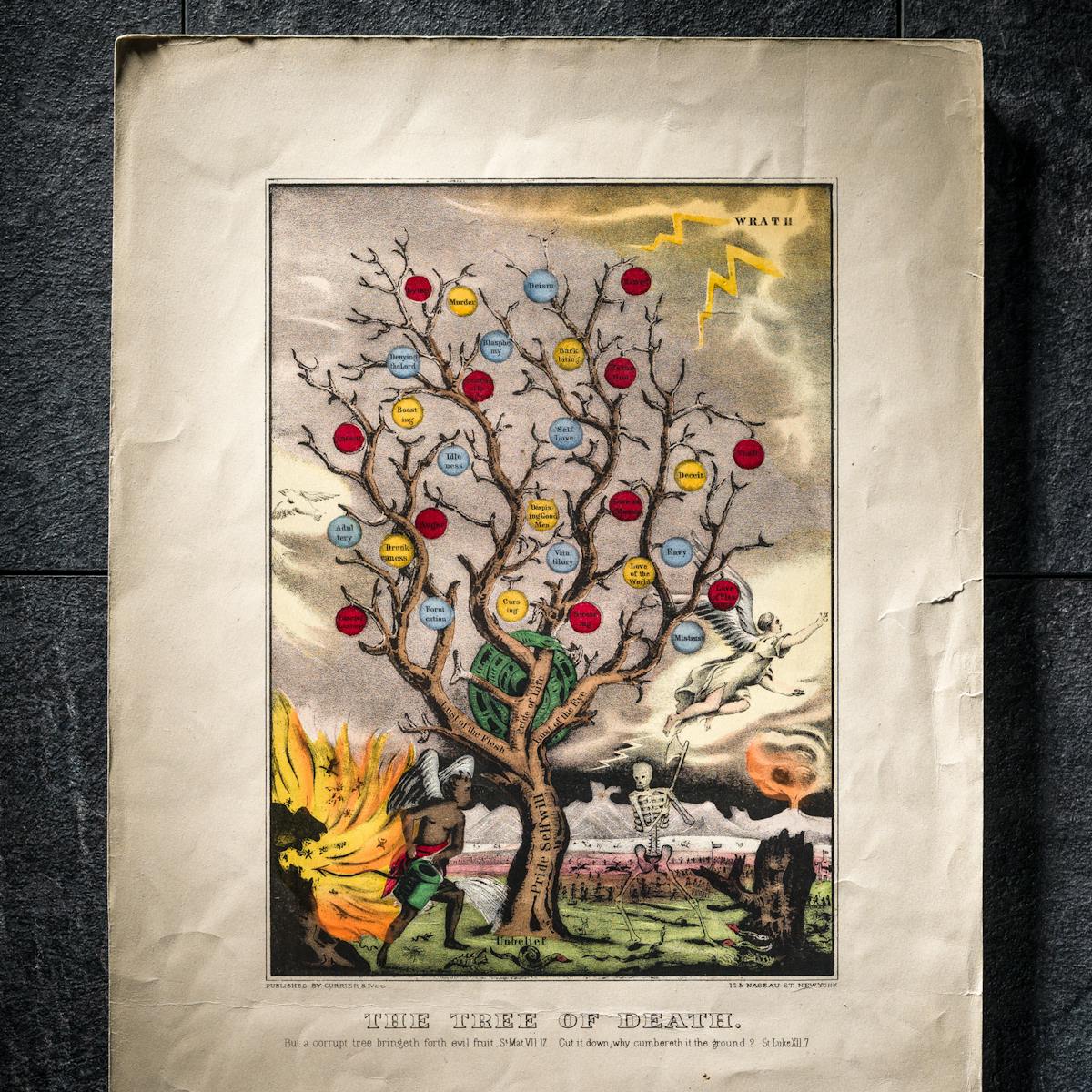The poster, titled "The Tree of Death," depicts an aged, yellowed piece of paper with a vertically-oriented rectangular illustration. At its center stands a leafless, brown tree with a thick trunk and multiple branches extending more vertically than horizontally. This tree bears hanging ornaments in blue, yellow, and red, each labeled with negative emotions or practices such as deceit, envy, and adultery. Above the tree, thunderclouds labeled "Wrath" release lightning bolts into the sky. At the base of the tree, a skeleton wielding an axe seems poised to cut it down, while to the left, a dark-skinned figure with black and white wings waters the tree. An angel can be seen flying in the background, and a cityscape and fire are visible towards the left of the image. The outlined letters at the bottom of this weathered paper frame the ominous title, "The Tree of Death."